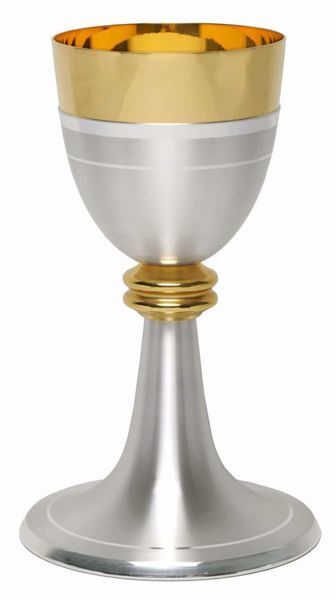This color photograph features a detailed depiction of an ornate chalice, often used in religious ceremonies such as those in a Catholic church. The chalice, crafted from two distinct metals, exudes both elegance and ceremonial reverence. Its base is fashioned from a shiny silver or brushed aluminum, broadening out in a circular fashion as it descends. Encircling this base is a thin, matte silver band that contrasts beautifully with the reflective quality of the rest of the base. 

Moving upward, the chalice features two gold disc-shaped connectors, reminiscent of large washers, which join the stem to the goblet part, adding a touch of regal opulence. The lower half of the goblet is also composed of the same shiny silver or brushed aluminum, adorned with two horizontal white stripes—a broader one near the middle and a narrower one closer to the base.

The upper portion of the goblet transitions into a lustrous orange hue, highlighted with subtle black accents. The lip of the chalice is capped with a striking shiny gold band, accentuating the vessel's elegance. 

Set against a stark white background, the chalice stands out, its untarnished and polished finish suggesting it is new and well-maintained. This detailed and visually striking chalice, with its intricate mix of metals and thoughtful design, emphasizes its likely role in solemn ceremonies, perhaps used for holding wine during communion.